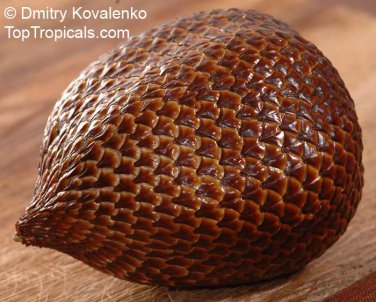The image is a close-up photograph of a tropical fruit, possibly a seed pod, set on a light brown, scratched wooden table. The photo itself is small and slightly rectangular, measuring about two inches high by two and a half inches wide. The fruit is distinctive with its armadillo-like scales, each dark brown in the center with a lighter brown edging. The scales grow larger and more pronounced from the narrow, pointed end where the stem would be, extending towards the bulbous right-hand side, giving the fruit a textured and dimpled appearance. In the top left corner of the image, © Dimitri Kovalenko and toptropicals.com are printed in white letters.